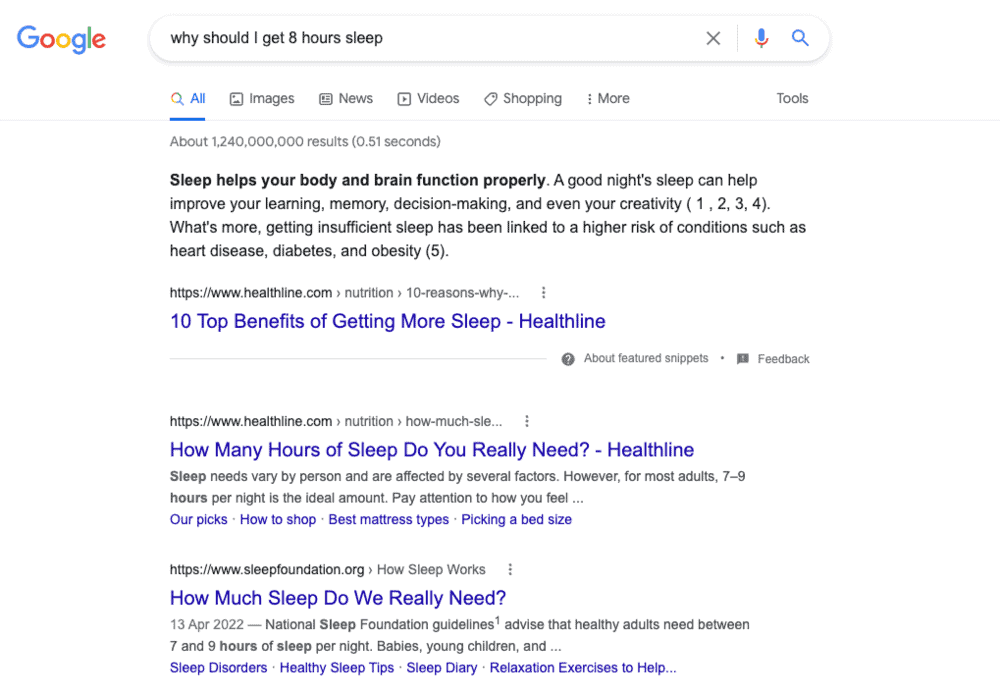This screen capture depicts a Google search results page. The URL at the top is not visible, but the iconic multi-colored Google logo is prominently displayed on the left-hand side. To the right of the logo is the familiar elongated search bar with a white background, blending seamlessly with the page's white backdrop. Inside the search bar, the user has entered the query: "why should I get eight hours sleep." On the right side of the search bar, there is a small black "X" icon for clearing the text.

Outside the search bar, you'll notice a colorful microphone icon, indicating the voice search option, and a classic blue magnifying glass, the search button. Below these icons, the word "Tools" is featured.

Directly beneath the search bar, the primary navigation menu of Google is displayed. The word "All" is highlighted in blue, showing it is the selected tab, with a blue line underneath it. Following this are icons and labels for other types of searches: Images (a photo icon), News (a newspaper icon), Videos (a video camera icon), Shopping (a tag icon), and a "More" option, separated by a vertical pipe sign.

It is also noted that the search returned approximately 1,240,000,000 results in just 0.51 seconds. 

The first search result starts with a bolded black header: "Sleep helps your body and brain function properly," from Healthline.com. Below the URL, in blue text, is the title "10 Top Benefits of Getting More Sleep | Healthline."

A grey divider line separates this from the second result, which also comes from Healthline, with the title in dark blue: "How Many Hours of Sleep Do You Really Need? | Healthline," followed by a brief snippet of text providing information about sleep.

The final notable search result is from the Sleep Foundation, with a black URL. The title in blue reads: "How Much Sleep Do We Really Need? | Sleep Foundation." This result also includes a paragraph of preview text, concluding with several blue-colored links: "sleep disorders," "healthy sleep tips," "sleep diary," and "relaxation exercises to help."

This descriptive view encapsulates the detailed layout and key elements of the search results page.